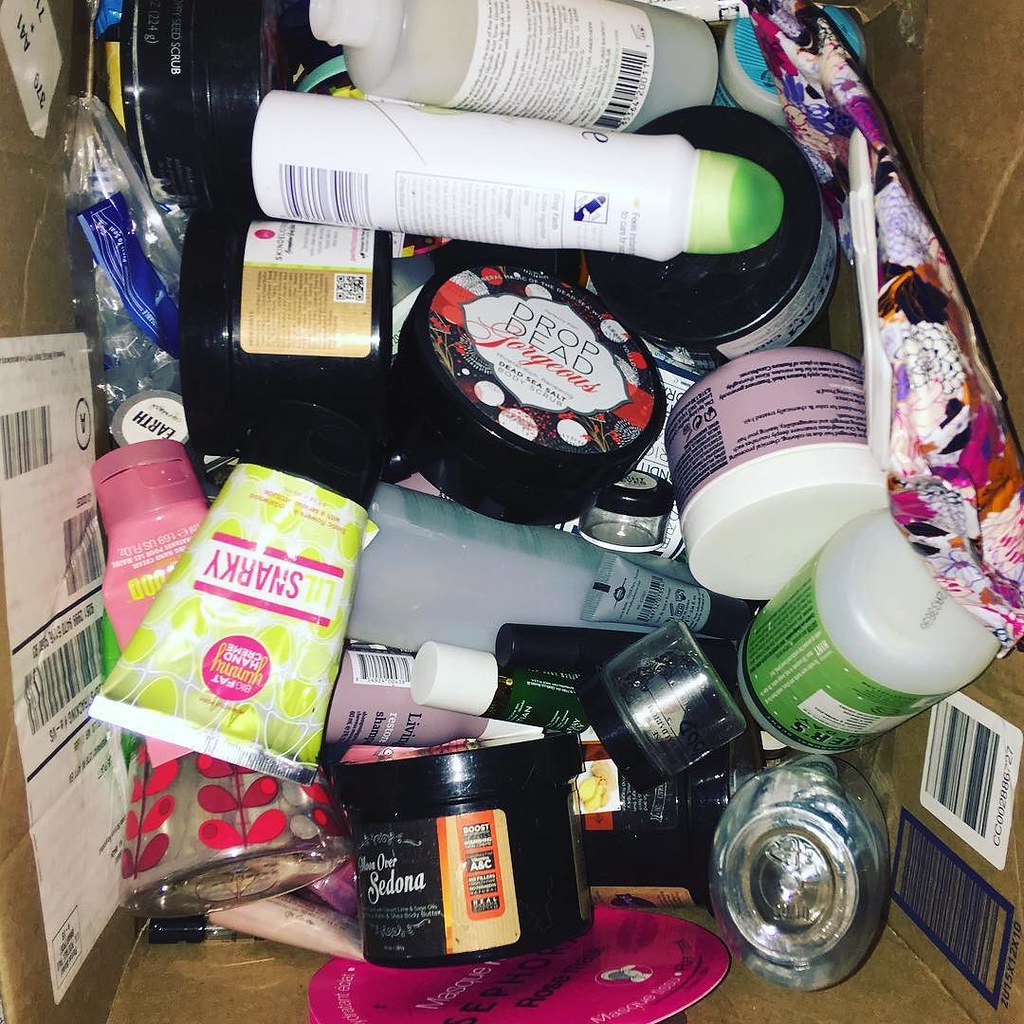This photograph captures an open cardboard box, with its sides forming the borders of the image. The box appears to be a haphazard collection of beauty and toiletry supplies, offering a peek into a chaotic stash of personal care items. Dominating the center of the box is a plastic bottle labeled "Drop Dead Gorgeous" in bold black font. Surrounding it are numerous black plastic jars, all contributing to the cluttered ensemble.

In the upper right corner, there's a translucent plastic toiletry bag adorned with a floral print and sealed with a white zipper. Scattered throughout the box are small plastic tubes, likely containing sunscreen and foundation. In the lower right corner, a few upside-down glass perfume bottles add a touch of elegance to the otherwise disorganized scene.

It seems as though an entire beauty shelf has been unceremoniously dumped into the box, creating a fascinating, albeit messy, snapshot of someone's personal care collection.